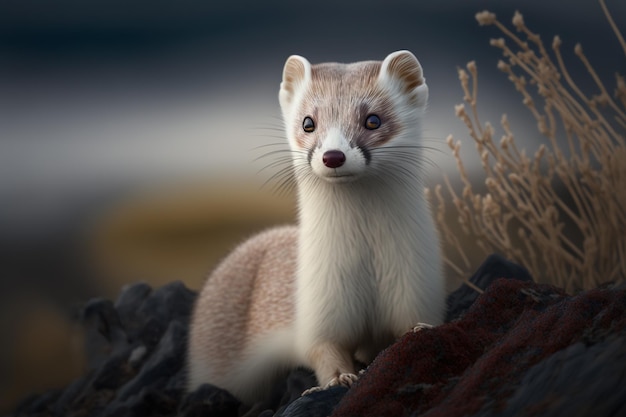The image is a highly detailed digital illustration, likely created by artificial intelligence, depicting an ermine or ferret-like creature centered in the composition. The animal has predominantly white fur on its chin and chest, and beige fur on its forehead and back. Its dark whiskers protrude prominently from its face, adding to its curious expression as it looks slightly off to the left of the viewer. The ermine has small, rounded ears, a pointed nose with a white snout, and rounded black eyes that seem somewhat out of place, hinting at its artificial origins.

The creature is positioned behind a boulder-like structure made of dark gray rocks, giving the impression that it is peeking out or hiding. To the right of the animal, there is a plant without leaves but adorned with tiny flowers at the top, and a cluster of beige dead grass. The background of the image is deliberately blurred, featuring dark blue and white hues that provide a sense of depth and focus on the subject. The overall style mimics wildlife or nature photography, though the illustration's artificial elements are subtly evident.